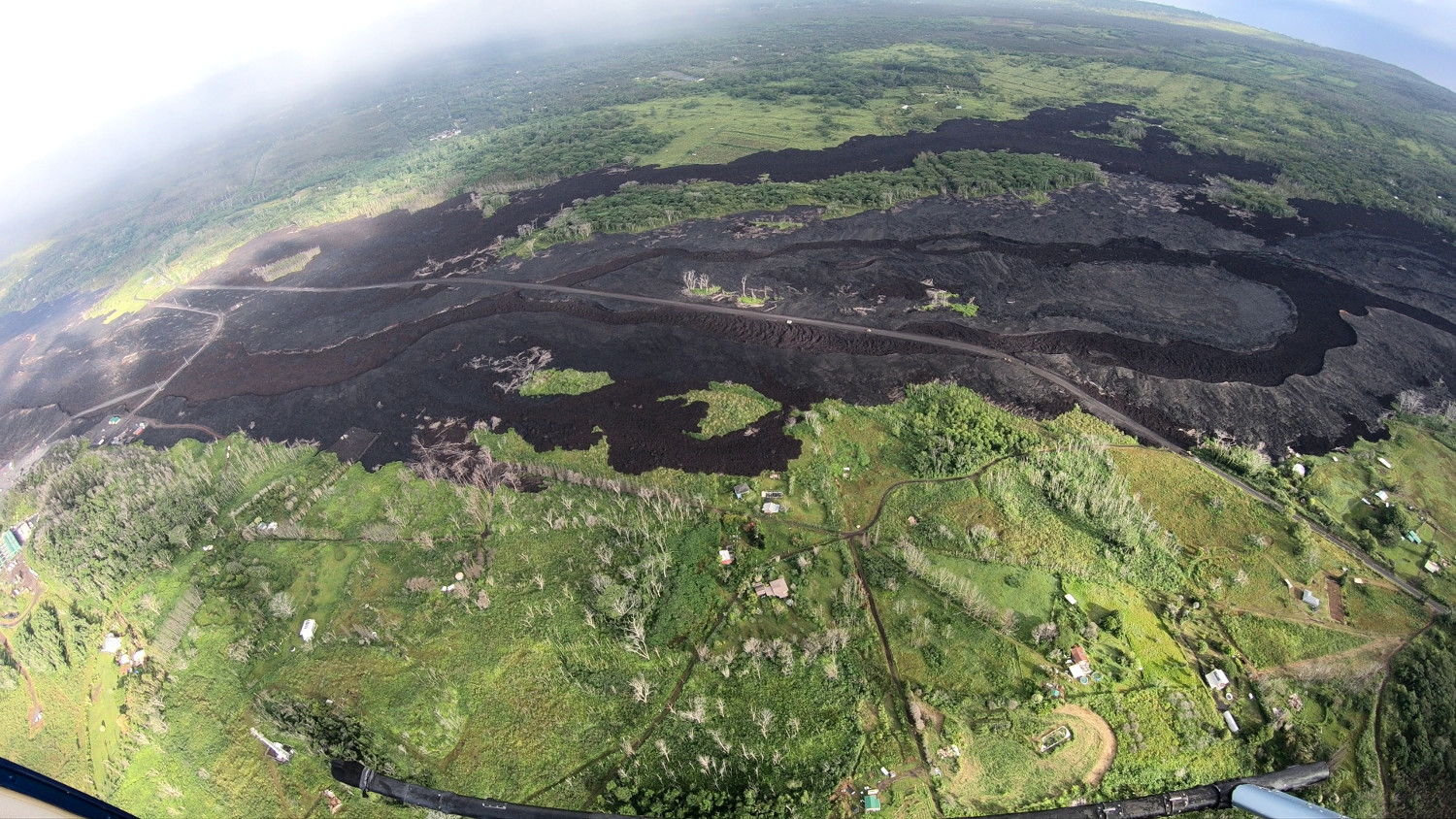This aerial photograph, likely taken from a helicopter, offers a sweeping view of a vast landscape consisting predominantly of green farmlands and intersecting roads. Positioned in the middle, several farms — a total of about five — are distinctly sectioned off, with each plot surrounded by a road network. You can detect various structures on the ground, including scattered houses, mostly white with red roofs, and some trees or shrubs dotting the greenery. A prominent feature is a large, contiguous area of dark soil or potentially cooled lava, suggesting significant land alteration — possibly for an upcoming freeway, as indicated by visible bulldozers and construction equipment. The image, distorted by a fish-eye lens, also captures the skids of the helicopter at the bottom, adding a sense of depth and perspective to the high-altitude view.